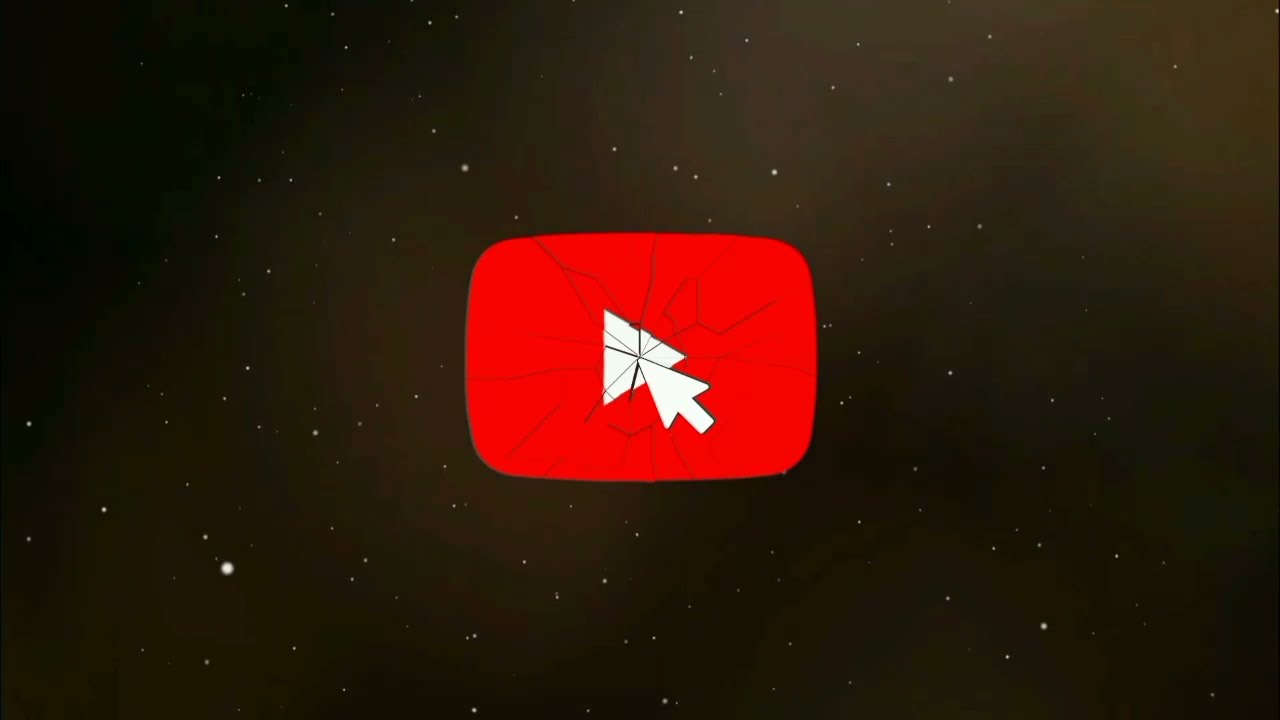The image showcases a digital representation with a striking black background, adorned with small white specks that evoke the appearance of a starry night sky. At the center, a conspicuous YouTube logo is prominently displayed. The logo is depicted as a red rectangle with rounded corners, featuring a white play button in its center. Over this emblem, a white mouse cursor hovers, positioned as if ready to click. A notable feature of the image is the cracked appearance of the YouTube logo; black lines radiate from the spot directly beneath the cursor, giving the impression of shattered glass. The overall aesthetic conveys a sense of disruption or impact, suggesting either a metaphorical breaking of the internet or highlighting a significant moment, such as the release of a pivotal video.